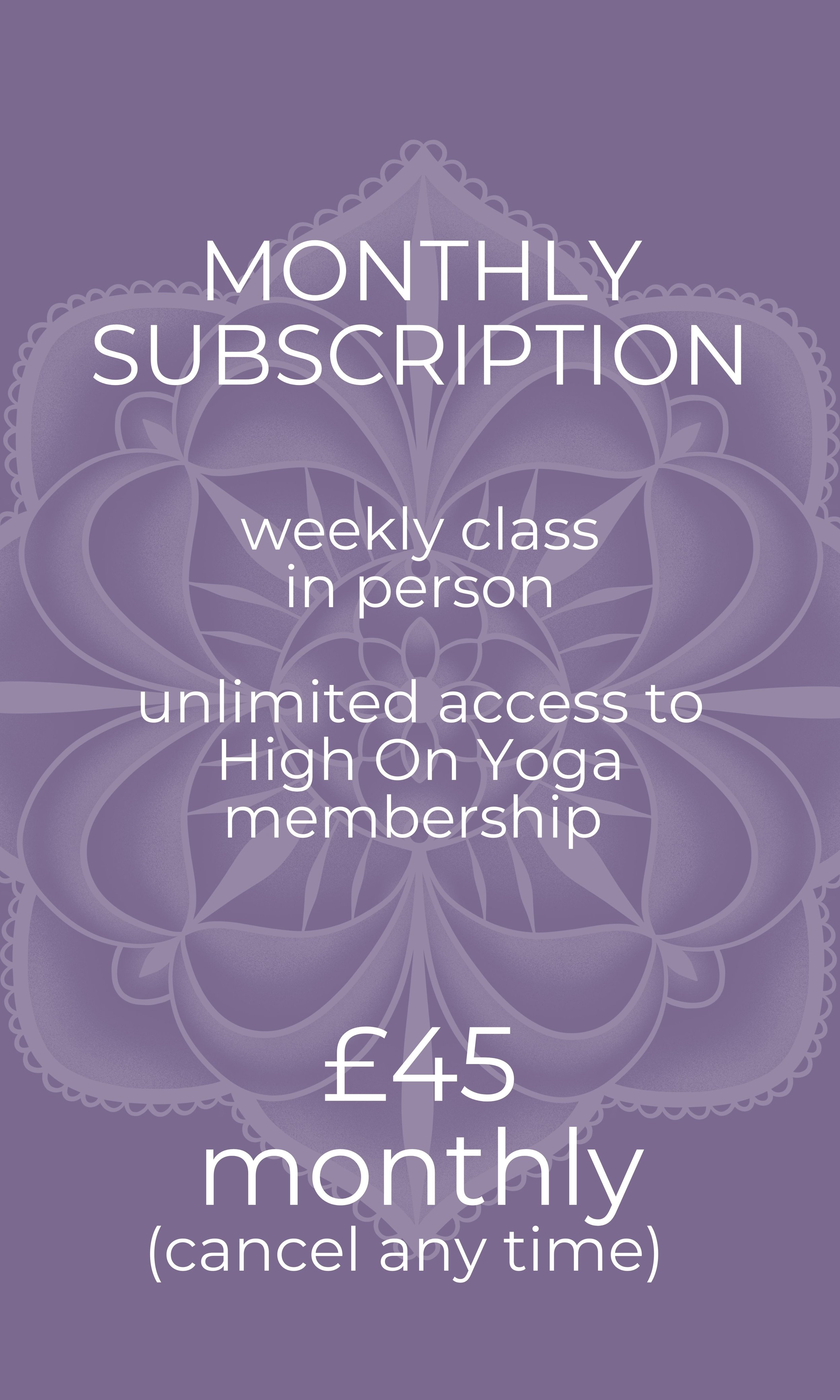Vertical rectangular image with a violet background featuring a delicate, ruffled flower design in light purple and violet tones. At the top center, the text "Monthly Subscription" appears in white, followed by "Weekly Class In Person." Below this, an additional text section reads "Unlimited Access to High-On Yoga Membership." Further down, a pound symbol (£) is displayed with "45" next to it, indicating the cost of the membership at £45 monthly. At the bottom in parentheses, it states, "Cancel at any time."